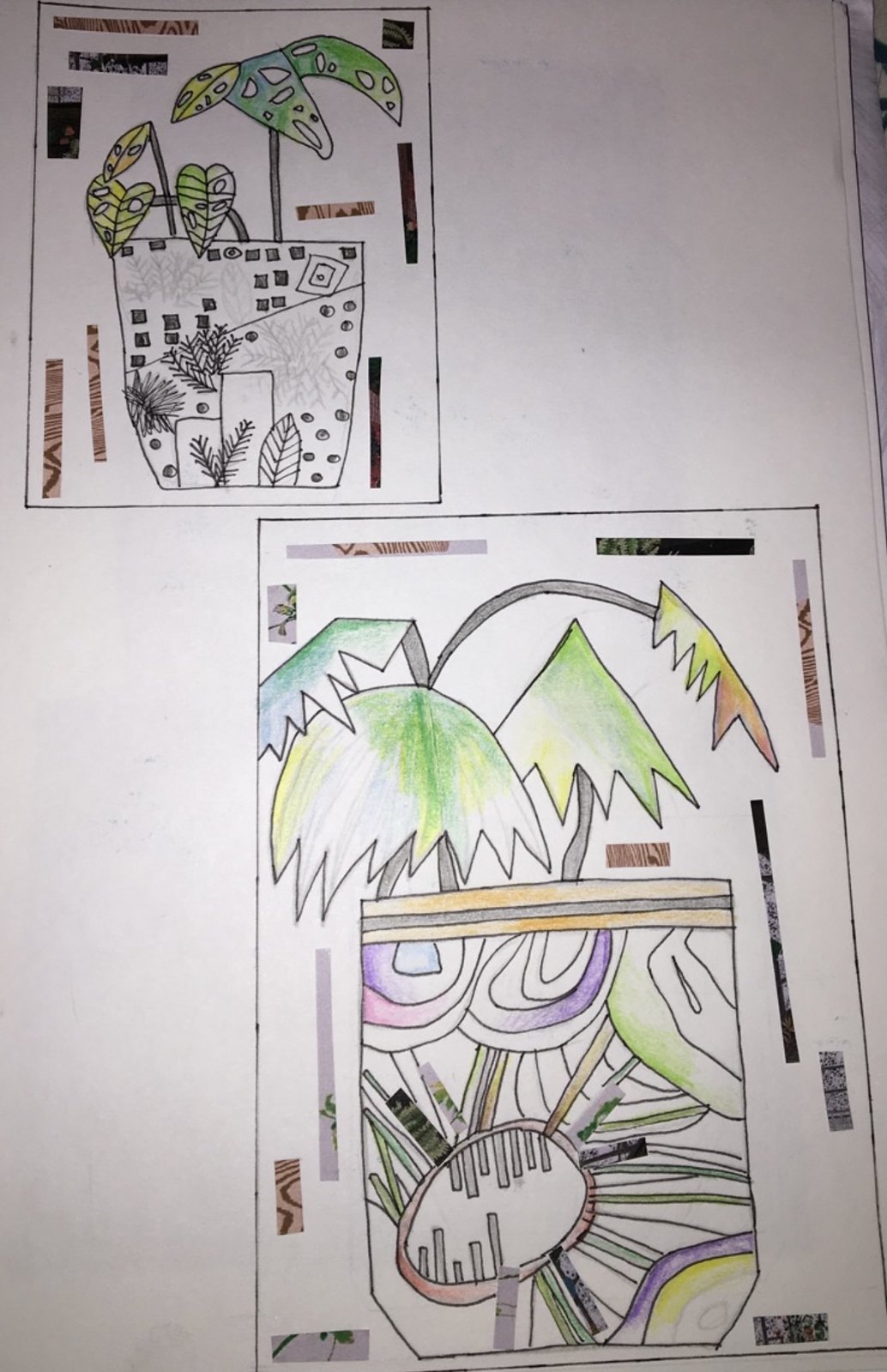This image features two distinct yet complementary pieces of art displayed on a single large sheet of paper. Both pieces are pencil sketches accentuated with colored pencils and bordered with small rectangular fabric swatches meticulously pasted around the edges, adding a tactile and decorative dimension. The artworks evidently depict planters with various plants, showcasing an intriguing blend of abstract and botanical elements.

The upper left drawing is relatively smaller, illustrating a black-and-white vase adorned with geometric shapes including squares and circles. Emerging from the vase are intricate representations of leaves and flowers, peppered with abstract shapes and dots. Notably, three smaller rectangular shapes with dots are positioned at the base of the vase, giving a layered texture to the composition. The leaves and floral elements are detailed with delicate lines and patterns, adding to the artwork's overall whimsical charm.

In contrast, the bottom right drawing is larger and predominantly colorful, featuring a somewhat rectangular pot with rounded lower edges. It boasts a vibrant mix of blue, purple, pink, and yellow circular designs resembling lollipops, which could be interpreted as abstract flowers. Stems in shades of brown branch out from the vase, supporting leaves with jagged edges that are colored in green, yellow, and orange. The depiction of stems and flowers here is more vivid, with distinctive colors and forms suggesting a playful, imaginative approach. Both artworks share a common theme of planters with plants, yet each piece brings its own unique aesthetic, making the entire composition a delightful exploration of artistic expression.